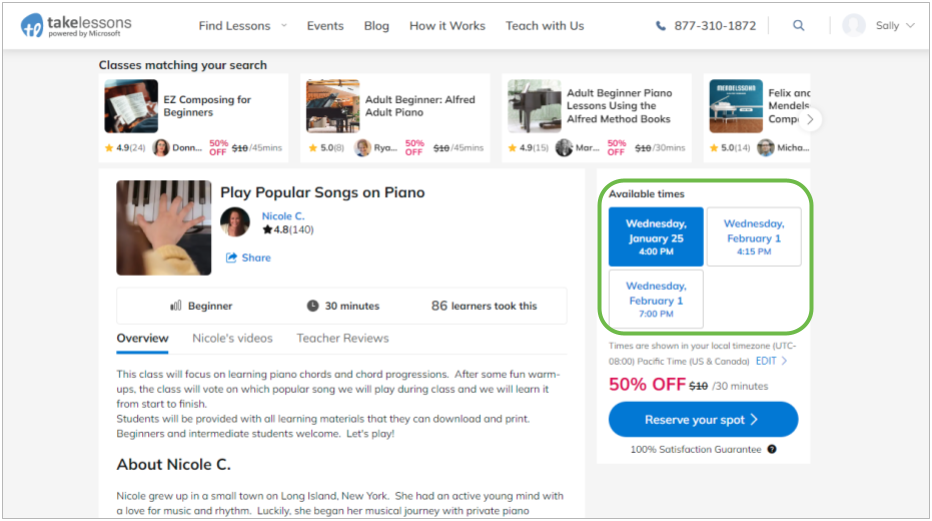This screenshot features a webpage with a light gray background. At the very top, a white bar stretches across the width of the page. In the upper left corner of this bar, there is an icon featuring a blue oval with white cursive letters "TL" at its center. Adjacent to the icon, in black font, are the words "Take Lessons, powered by Microsoft."

To the right of this text, there is a drop-down menu labeled "Find Lessons." Following that, there are links for "Events," "Blog," "How It Works," and "Teach Us." Further along, there is an icon shaped like a phone handset next to the phone number 877-310-1872. To its right, there is a magnifying glass icon representing a search function, followed by a small circle with a white silhouette of a human. Next to this icon, the name "Sally" is displayed along with a drop-down menu.

Directly beneath this header, the webpage content begins. At the top of this section, there are four white squares arranged horizontally, each labeled "Classes Matching Your Search." The first square on the left is titled "Easy Composing for Beginners." Next to it is a square labeled "Adult Beginning, Alfred Adult Piano."